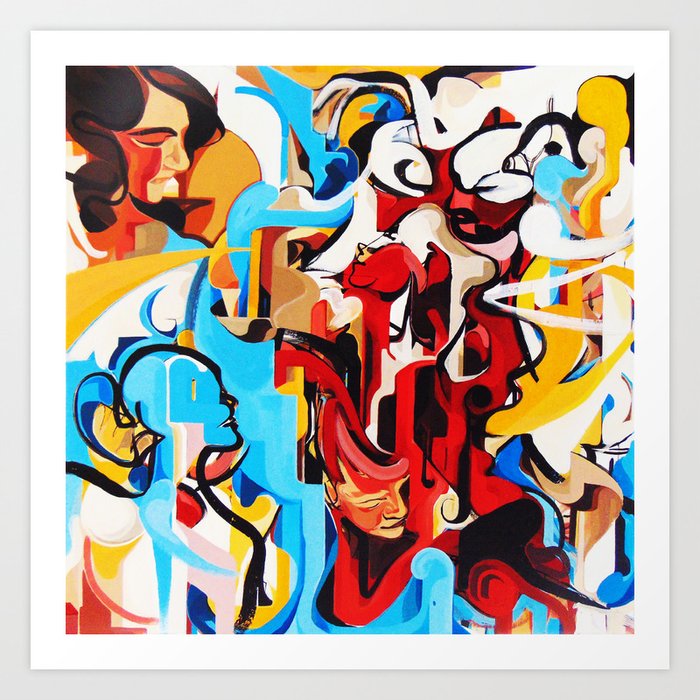This abstract painting, set within a thick white border and framed on a white background, bursts with vibrant and bold hues of bright blue, red, yellow, brown, orange, white, and black. The composition is intricate, filled with a mix of circular shapes, sharp angular lines, and energetic movements. In the upper left corner, there is a prominent stylized portrait of a woman with brown hair, red accents on her face, and white skin, gazing downward with a slight smile. Below her, in the bottom left corner, a black silhouette of another woman, featuring her outline and visible hair and breasts, looks up to the right. Amidst the colorful swirls and shapes throughout the painting, numerous profiles of faces and silhouettes of women emerge, adding depth and complexity to the vibrant abstract scene.